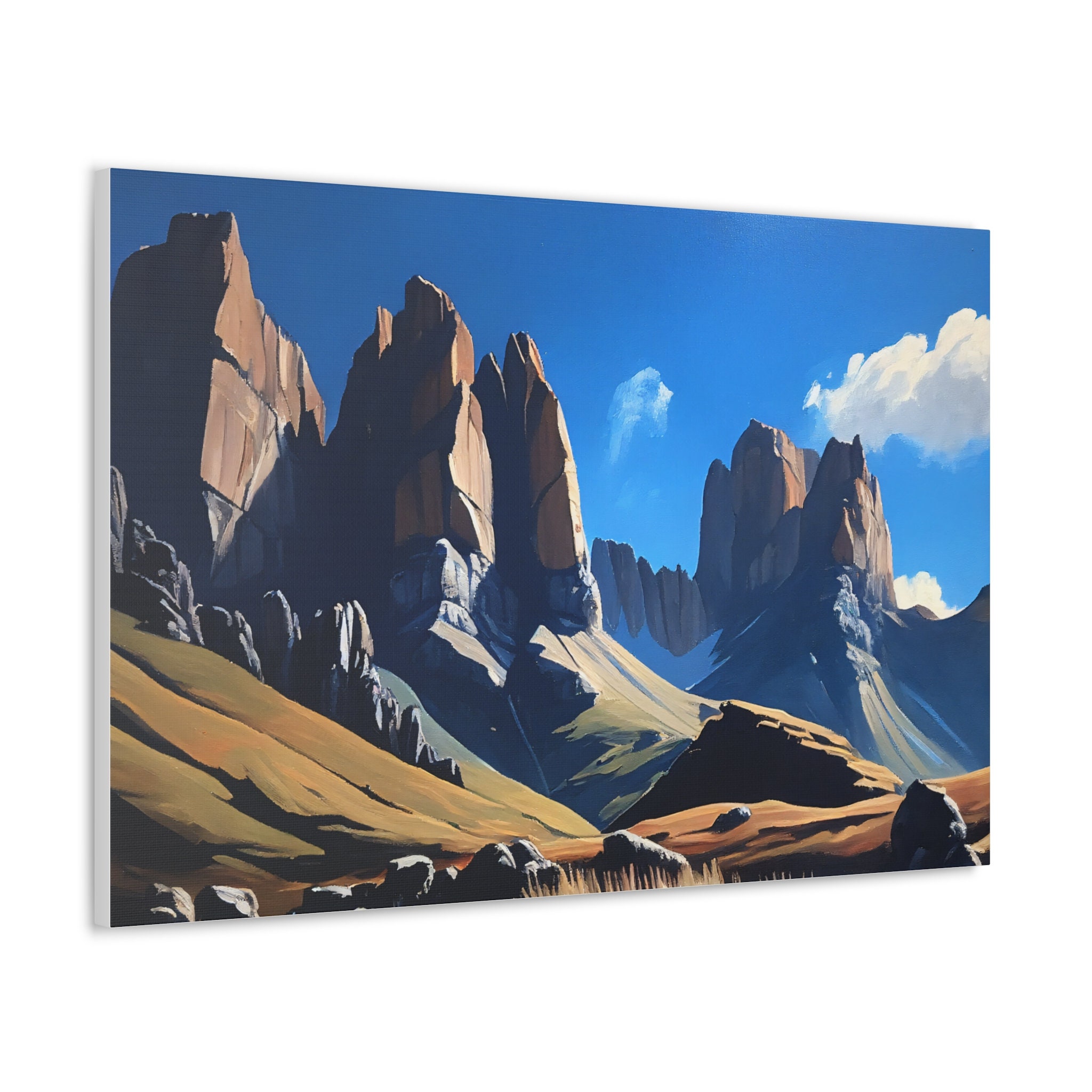This cartoonish-style painting depicts a vivid landscape resembling the canyons and mountains seen in Wyoming and Utah. Dominated by a bright blue sky adorned with a few wispy white clouds, the scene features majestic, snow-dusted mountains in the background. The foreground showcases a canyon with reddish-brown, tan, and gray boulders interspersed with hints of yellow grass. The colors are varied, with the mountains and rocks exhibiting shades of brown, reddish-brown, and faint yellow, contrasting sharply with the vibrant sky. A slight picture frame on the left suggests that this piece could be a wall hanging or part of a gallery display, pointing to an AI-created artwork that blends realistic and cartoonish elements for a unique, visually engaging effect.